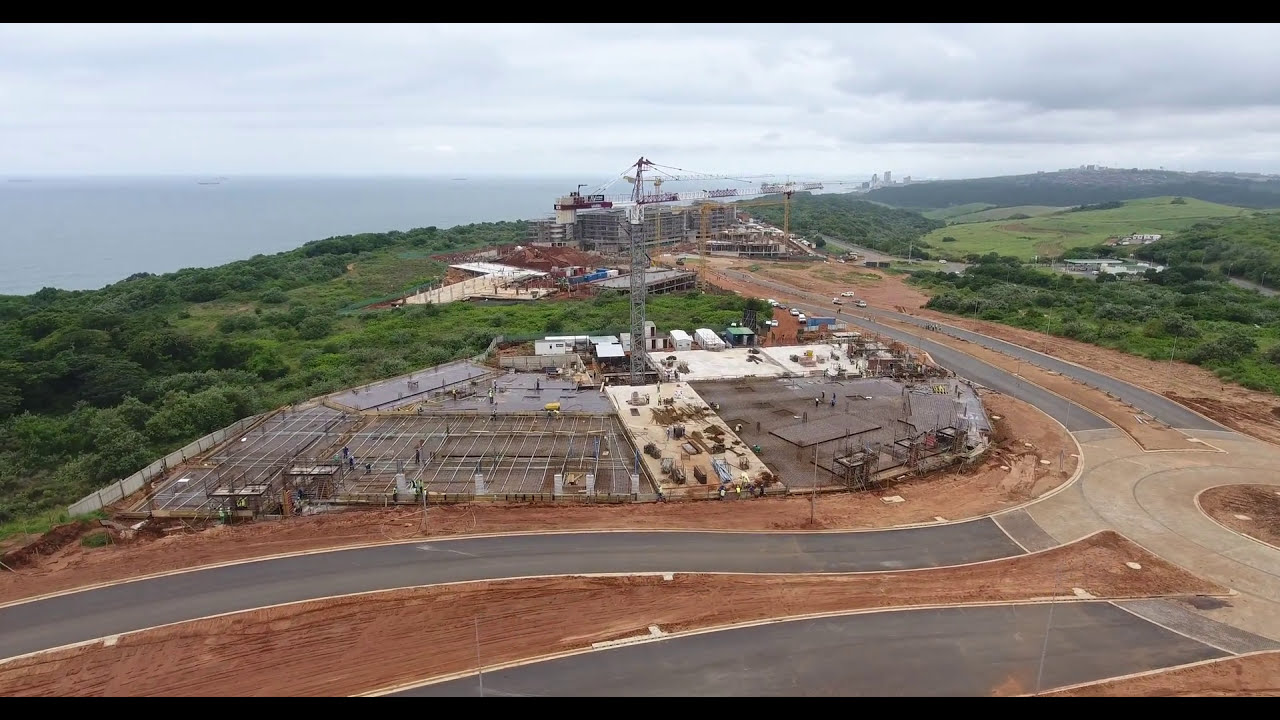The image is a horizontally rectangular, full-color photograph taken outdoors on an overcast day. Framed with a thin black border at the top and bottom, the image showcases a construction site with various elements. Starting from the left corner, a large body of water is visible, surrounded by a lush area of green plants, likely trees. The scene also features a brown dirt area interspersed with asphalt roadways winding and twisting across the frame. 

Central to the image, a roundabout converges multiple roads coming from different directions, including one extending from the bottom right up through the center. These roads surround an active construction site where two buildings are being erected. The structure in the background is further along, comprised mainly of girders, while the one in the foreground shows early stages of development with rebar laid out on the ground. Tiny construction workers can be seen if one looks carefully. The setting, under a cloudy sky, presents a palette of gray, brown, green, blue, tan, and shades of white, capturing a detailed and dynamic construction scene.